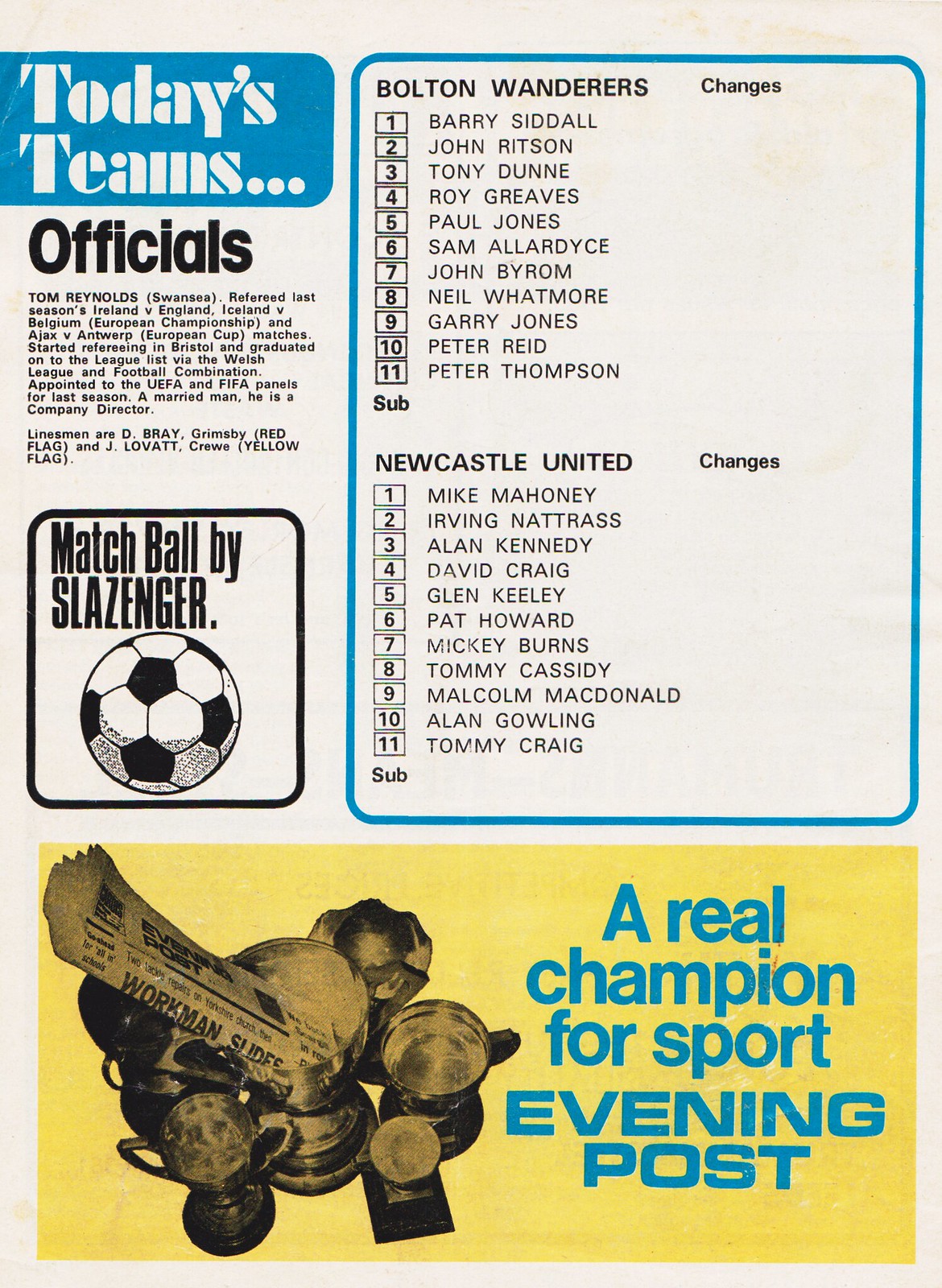This page, taken from a vintage UK football club guide, features a detailed layout of a soccer match between Bolton Wanderers and Newcastle United. At the top of the page, set against an aged white background with sections of blue and yellow, the heading "Today's Teams" is prominently displayed with the names of the players from both teams listed underneath. The Bolton Wanderers squad includes Barry Siddal, John Ritson, Tony Dunn, Boyd Greaves, Paul Jones, Sam Allardyce, John Byram, Dale Watmore, Gary Jones, Peter Reed, and Peter Thompson, while the Newcastle United lineup features Mike Mahoney, Irving Natras, Alan Kennedy, David Craig, Glenn Kealy, Pat Howard, Mickey Burns, Tommy Cassidy, Michael McDonald, Alan Gelling, and Tommy Craig.

Below the team listings, the page details the match officials. A noteworthy ad for a match ball by Schlesinger is mentioned both under officials and by the players' listings. The lower section of the page highlights a gold-tinted advertisement by the Evening Post, complete with a photograph of trophies surrounding a rolled-up copy of the newspaper, reinforcing the tagline "A real champion for sport." The page features mostly black text, with accents in blue and a faded pinkish-white background, all bordered by a yellow rectangle at the bottom, indicating its age. The entire layout, filled with historical elements, likely depicts an era gone by.